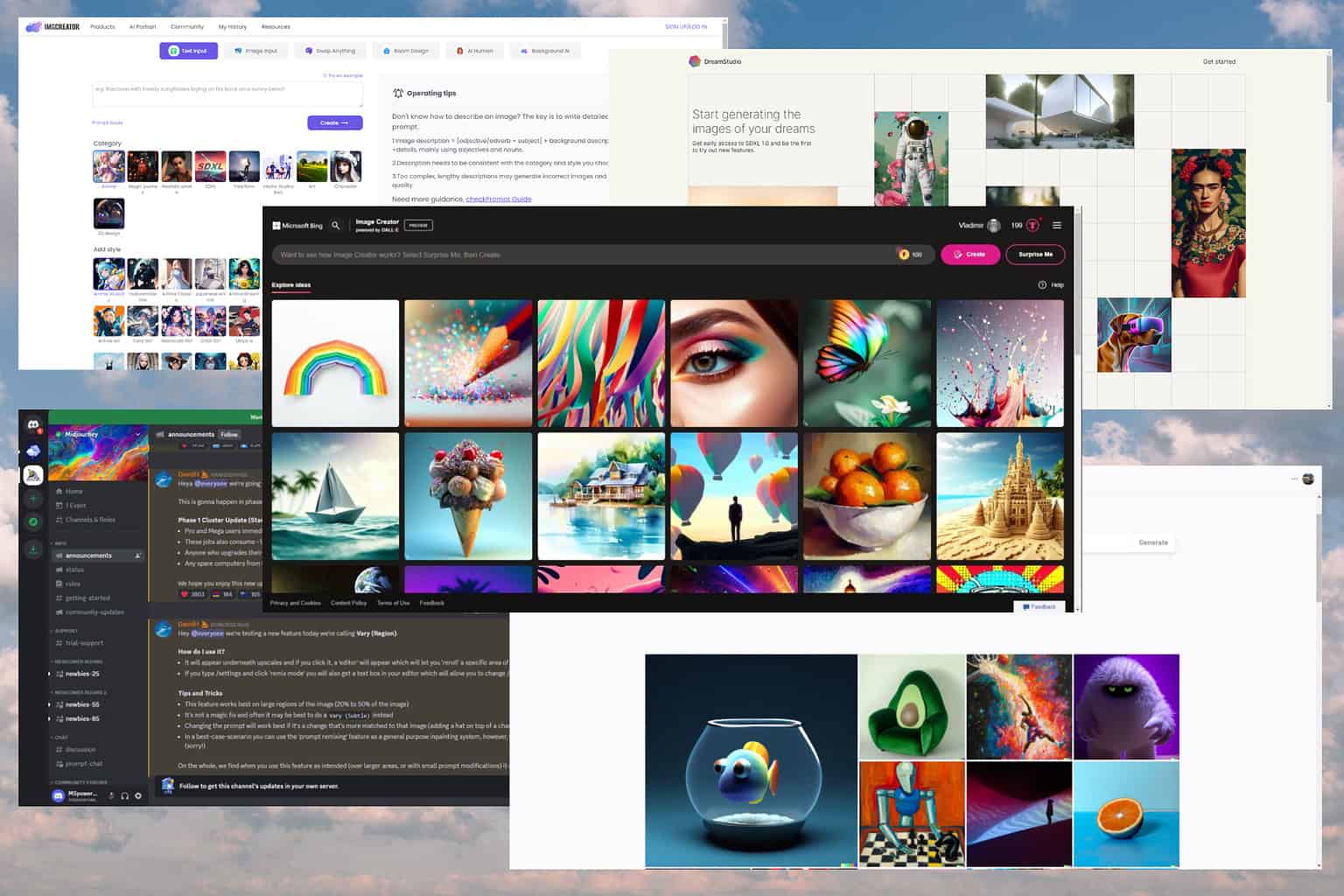This screenshot captures the interface of what appears to be a photo-storage or photo-sharing application. The screen is populated with multiple windows, each displaying a collection of high-quality photographs. The images within these windows showcase a variety of subjects, including vibrant fruits like avocados, colorful rainbows, delectable ice cream cones, and various other items. Additionally, some of the photographs feature female subjects. The array of windows and diverse imagery suggest that the app is used for organizing and viewing a wide assortment of photographic content.